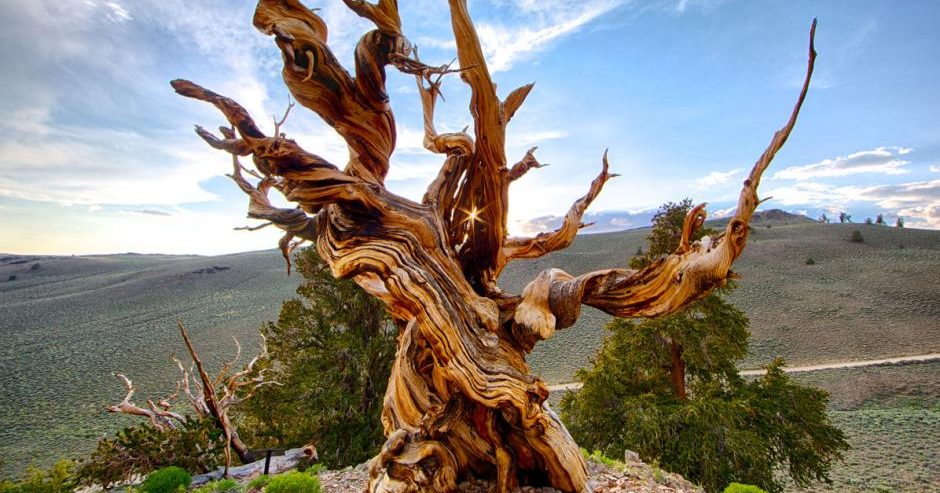The image captures a striking, solitary tree that stands prominently on top of a hill, or possibly a dune, against a backdrop of a barren landscape. This unique tree is characterized by its twisted and mangled trunk, which spirals and twists in various directions. The trunk is not uniform but features intricate color variations and jagged edges where branches have broken off. The immediate area around the tree is predominantly dirt with patches of greenery, including a couple of notably green bushes. Below the hill, the land is relatively flat and barren with very little vegetation, except for two trees that do have some greenery on their branches. There's a dirt road cutting through this desolate terrain. The sky is dotted with clouds, suggesting it might be around midday. The overall scene presents a stark and dramatic contrast between the twisted, almost creature-like tree and the sparse, desolate landscape. Additionally, there are a few people in the background, adding a touch of life to this otherwise deserted scene.